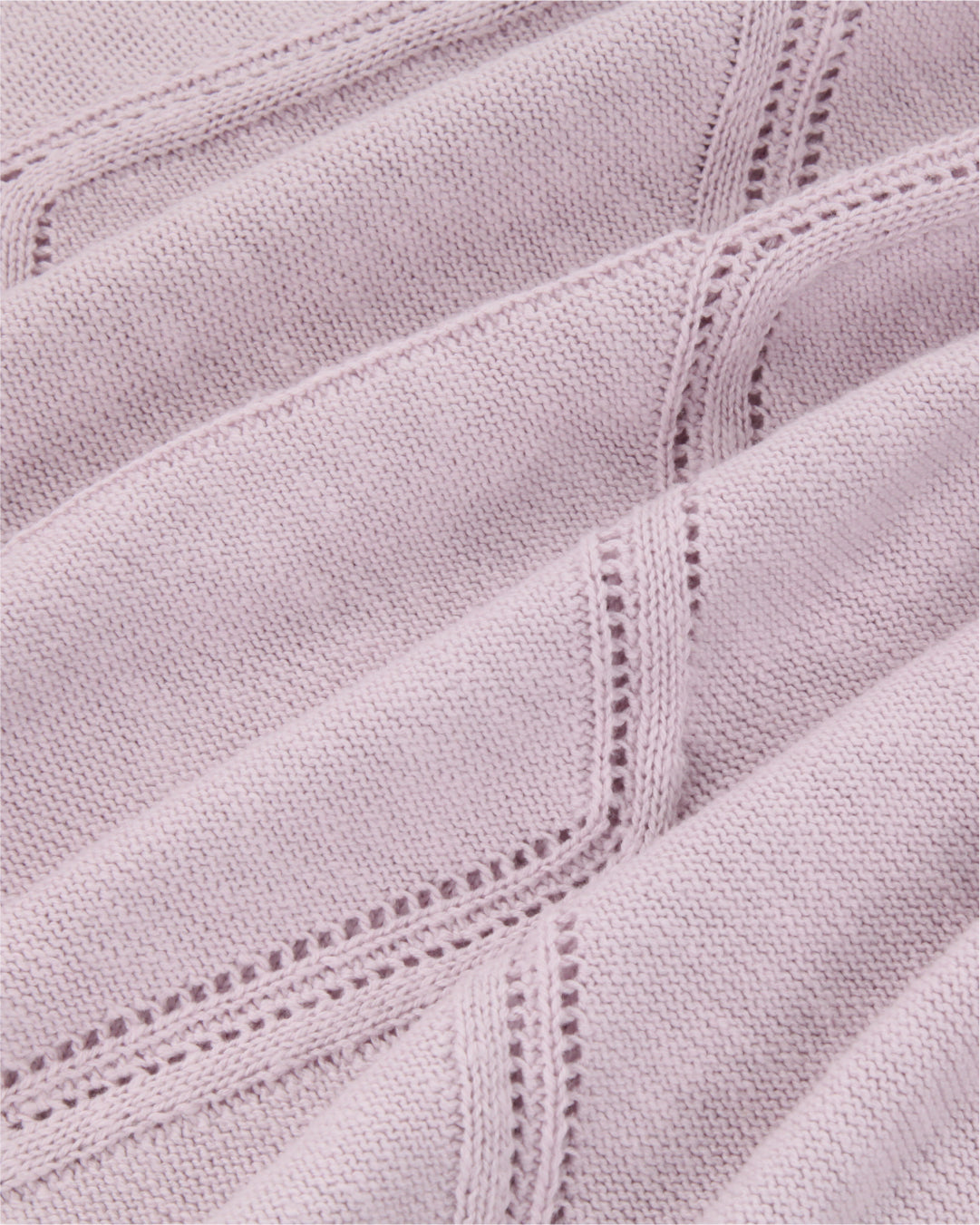This vertical, monochrome photograph features a light purple, knit fabric laid out flat, giving a soft and textured look. The fabric has small, intricate holes woven in repeating rows, creating a pattern of densely knitted sections interspersed with these larger holes. The knit is scrunched and pleated, forming undulating folds that extend from the bottom left to the top right. This detailed, close-up image showcases the delicate stitches and varying textures of the fabric, highlighting the darker purple stitching without any background distractions or text.